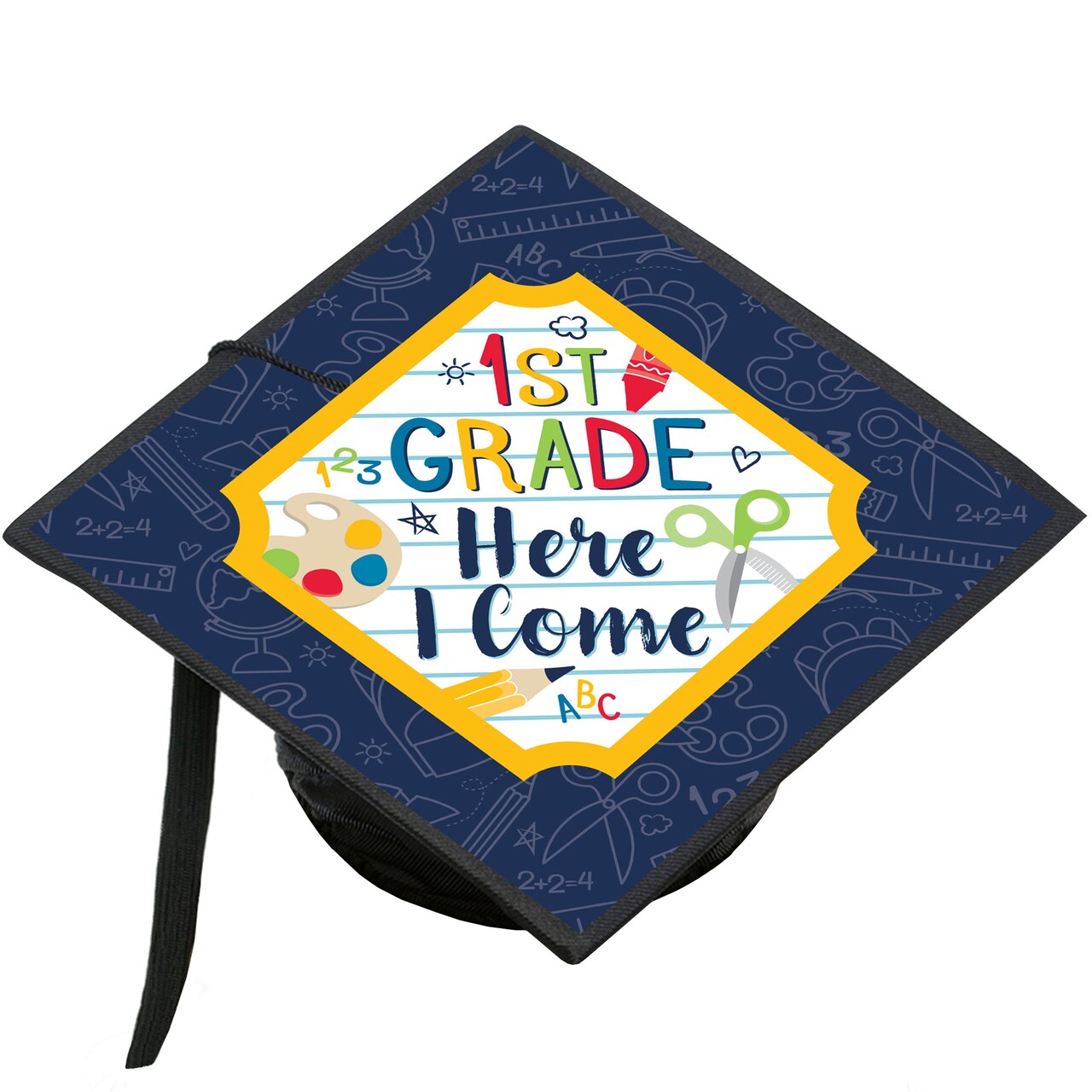The image depicts a computer-generated drawing of a kindergartner's graduation cap, viewed from above. The cap features a flat top with a vibrant and intricate design. The background of the cap is predominantly blue, adorned with line drawings of school-related items such as scissors, rulers, pencils, paint palettes, and mathematical equations like "2 + 2 = 4." 

At the center of the cap is a distinctive square with scalloped corners outlined in gold. The interior of this square has a white background with green lines, giving it a notebook-like appearance. Across this white background, in colorful letters of red, blue, green, and gold, the phrase "First Grade, Here I Come!" is prominently displayed. Surrounding the text within the square are various illustrations: a pair of green-handled scissors, a yellow pencil, a miniature paint set with primary colors (yellow, blue, red, and green), the alphabets "A, B, C," the numbers "1, 2, 3," a cloud, a heart, a star, and a sun. 

The cap, dark blue beneath the decorative top, includes a black piece of fabric hanging off the left corner, indicative of a graduation cap’s traditional tassel.